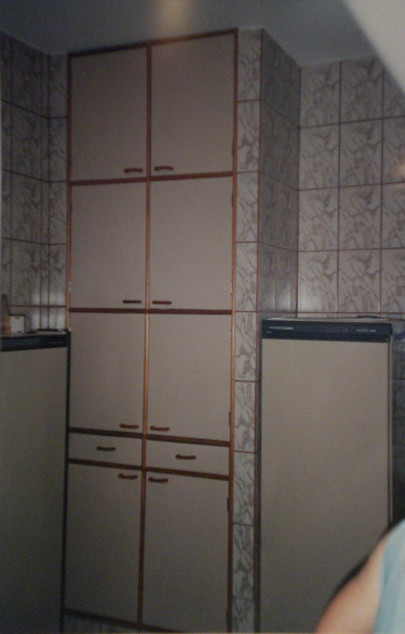This color photograph, taken in portrait format, captures a built-in floor-to-ceiling cabinet system inside an indistinct room of a house. The cabinets have three pairs of doors stacked vertically above a pair of drawers with two separate handles, followed by another pair of doors at the bottom. The cabinet doors and drawer faces are made of a solid light color framed by a coppery brown edging and feature plain horizontal handles. Surrounding the cabinets is a gridded wall covering with a marbled design, resembling white tiles with gray veins. In the lower right corner of the image, the blurred arm and shirt of a person are visible, adding a human element to the scene but offering no further clues as to the room's specific function.